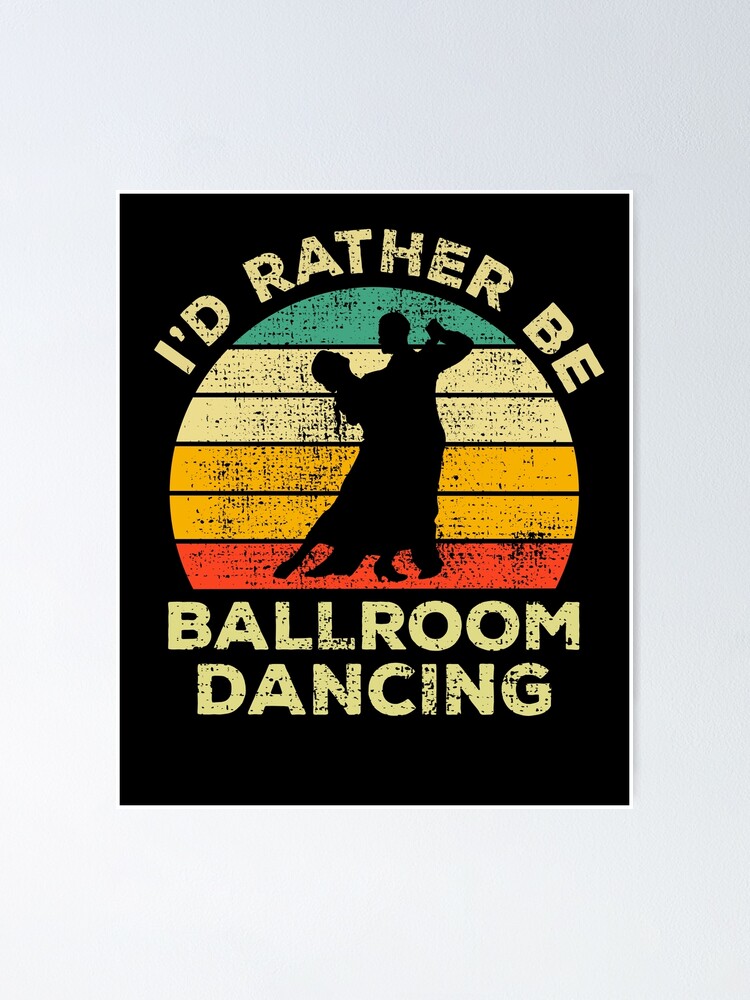This image features a gray background with bold, capitalized yellow text that reads "I'd rather be ballroom dancing." At the center of the image, a dynamic silhouette of a dancing couple is prominently displayed in black. The woman has her back arched gracefully, while the man holds her arm behind his shoulder, capturing a moment of elegant movement. 

Behind the couple, there is a semi-circular emblem featuring multiple colored stripes. Starting from the bottom, the stripes are red, followed by two dark orange, two cream, and finally, teal blue at the top. This composition suggests a vibrant, colorful backdrop that contrasts with the monochromatic figures, making the image pop. The overall aesthetic and the repeating message appear designed for dedicated ballroom dance enthusiasts, potentially as a unique t-shirt design that showcases a passion for dancing.